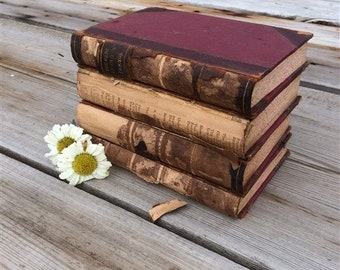This color photograph features a stack of four thick, old hardcover books sitting on a naturally textured wooden floor or deck outside. The wooden surface has an unpolished appearance, showcasing the wood's natural brown hue. The books are quite aged, with the spines starting to deteriorate and one book's spine nearly missing. A noticeable piece of one spine is broken off and lies beside the pile. The top book has a dark purple or mahogany brown cover, though the surface is peeling and shows signs of wear, resembling scorching. Adjacent to the books are two white flowers with large yellow centers, adding a delicate contrast to the scene.